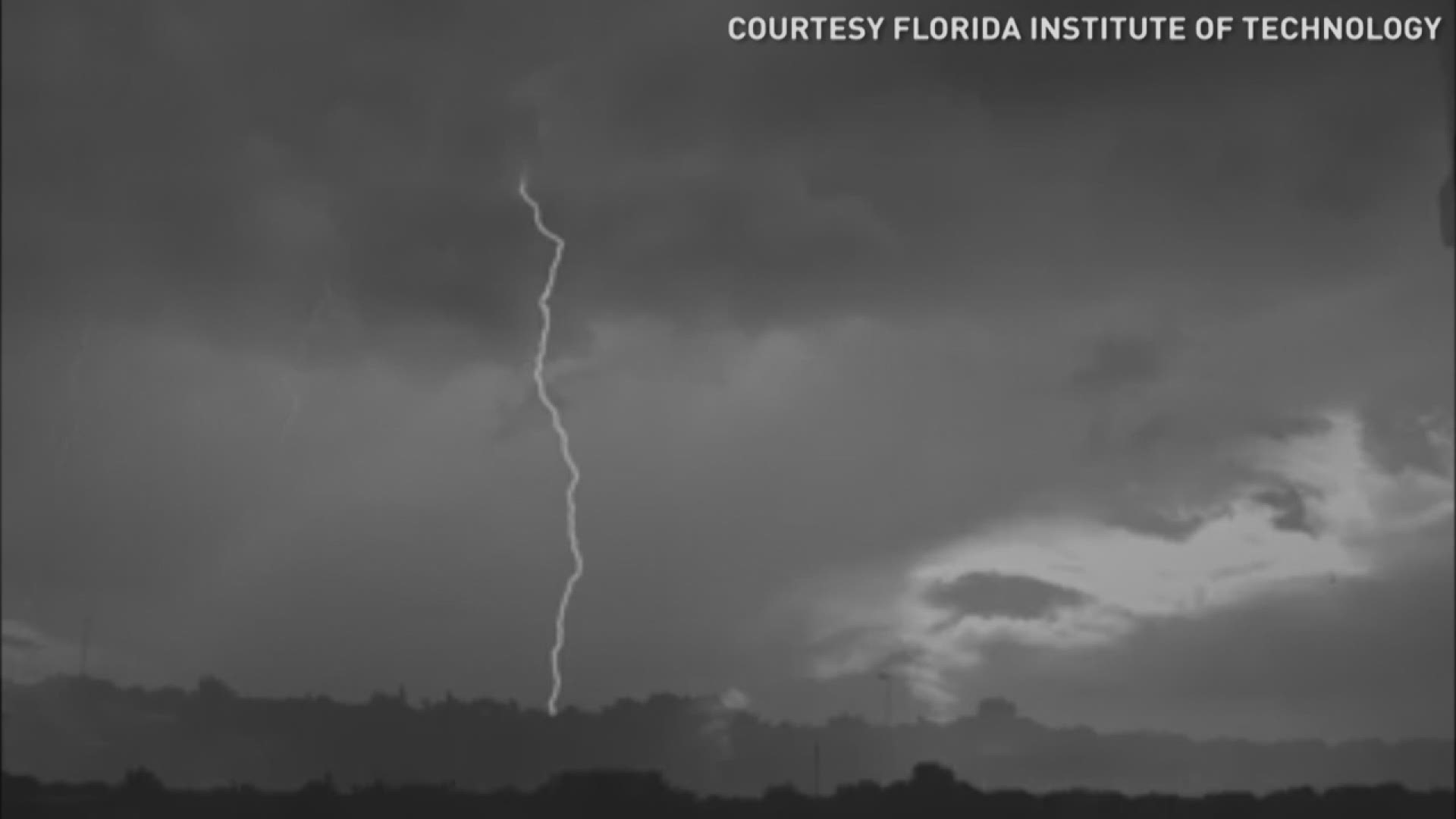This detailed black-and-white photograph captures the raw intensity of a powerful storm. Centered slightly to the left, a striking bolt of lightning pierces through the dark, tumultuous clouds, illuminating the scene with an electrifying flash. The sky is filled with various shades of gray, suggesting a fierce storm in progress. Toward the right side of the image, there is a notable gap in the clouds, possibly hinting at the parting of the storm or the formation of a tornado.

Framing the stormy sky is a silhouetted landscape featuring a tree-lined area and some vague shapes in the background that could either be mountains or additional trees, hard to distinguish due to the grayscale nature of the photograph. At the very bottom of the image, more darkened trees and possibly the faint outline of power lines or a village can be seen, blending into the almost monochromatic foreground.

Prominently inscribed at the top-right corner in white lettering is the credit, "Courtesy Florida Institute of Technology," ensuring viewers know the source of this dramatic imagery. The photograph is wider than it is tall and is devoid of any visible people, animals, buildings, or distinct man-made structures apart from the ambiguous power lines and possibly small structures at the bottom.